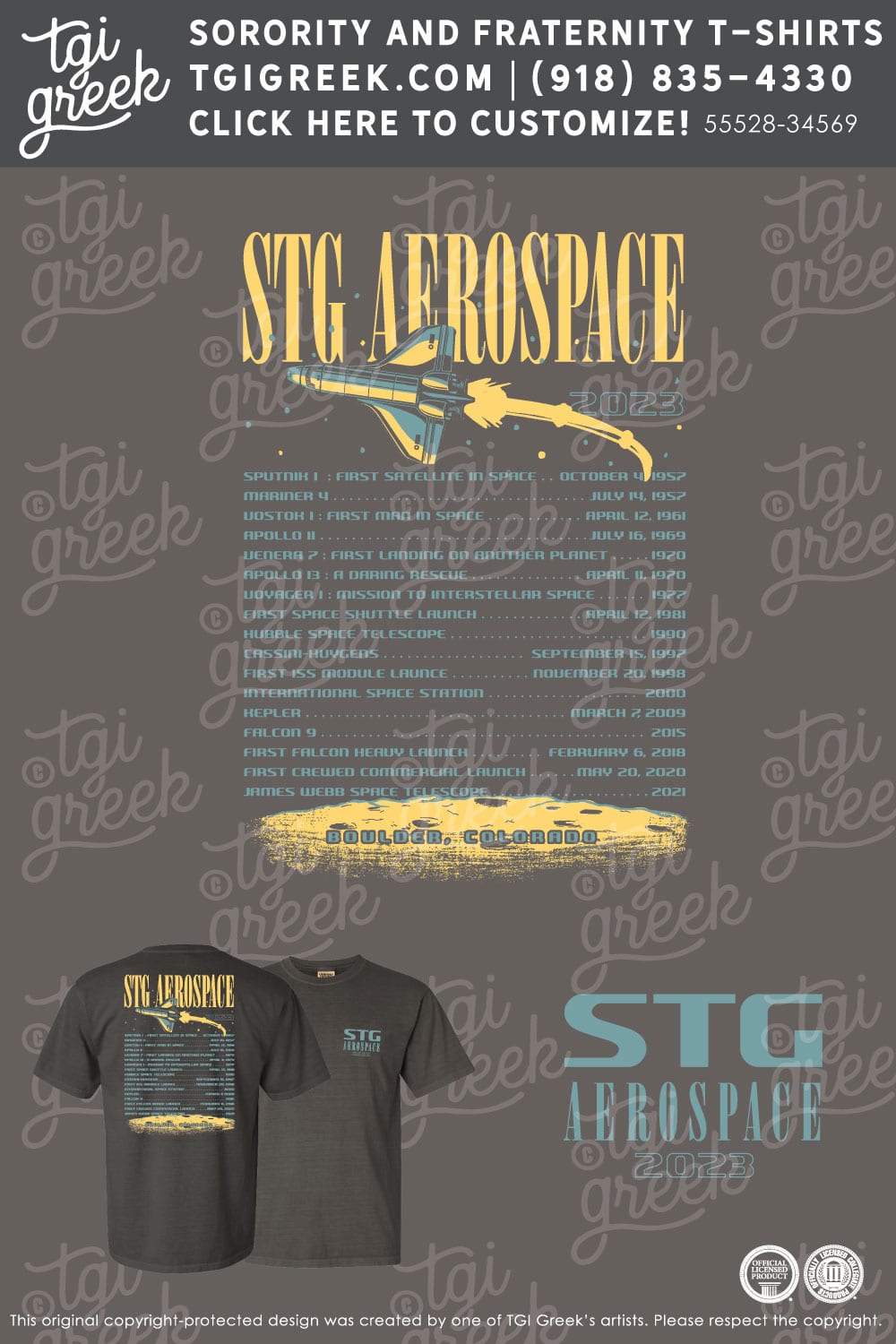This is an advertisement for customizable fraternity and sorority t-shirts by TGI Greek. At the top, there is a dark gray rectangular border about two inches high running the width of the page. On the left side of this border, "tgi greek" is written in white cursive letters, followed by "SORORITY AND FRATERNITY T-SHIRTS," "TGIGreek.com," and the phone number "918-835-4330" in capitalized, printed white font. Below this border, the background is a slightly lighter dark gray, featuring "STG Aerospace" written in yellow letters at the top, accompanied by an illustration of a yellow and blue rocketship soaring through the sky, with its trail visible. Beneath this, there appears to be a list of tour dates in blue text, formatted with city, state, venue name, and dates, though it's noted that the text isn't easily legible. On the bottom left corner of the ad, there are images of a black t-shirt showing both the front and back; the front displays the "STG Aerospace" logo in blue, and the back lists the tour dates. The same "STG Aerospace" logo is also seen on the bottom right corner of the ad. The entire image is overlaid with a light gray TGI Greek watermark, repeating throughout the background. Additionally, the ad includes customization details and a product number, with a note on the original design being copyright protected by TGI Greek.